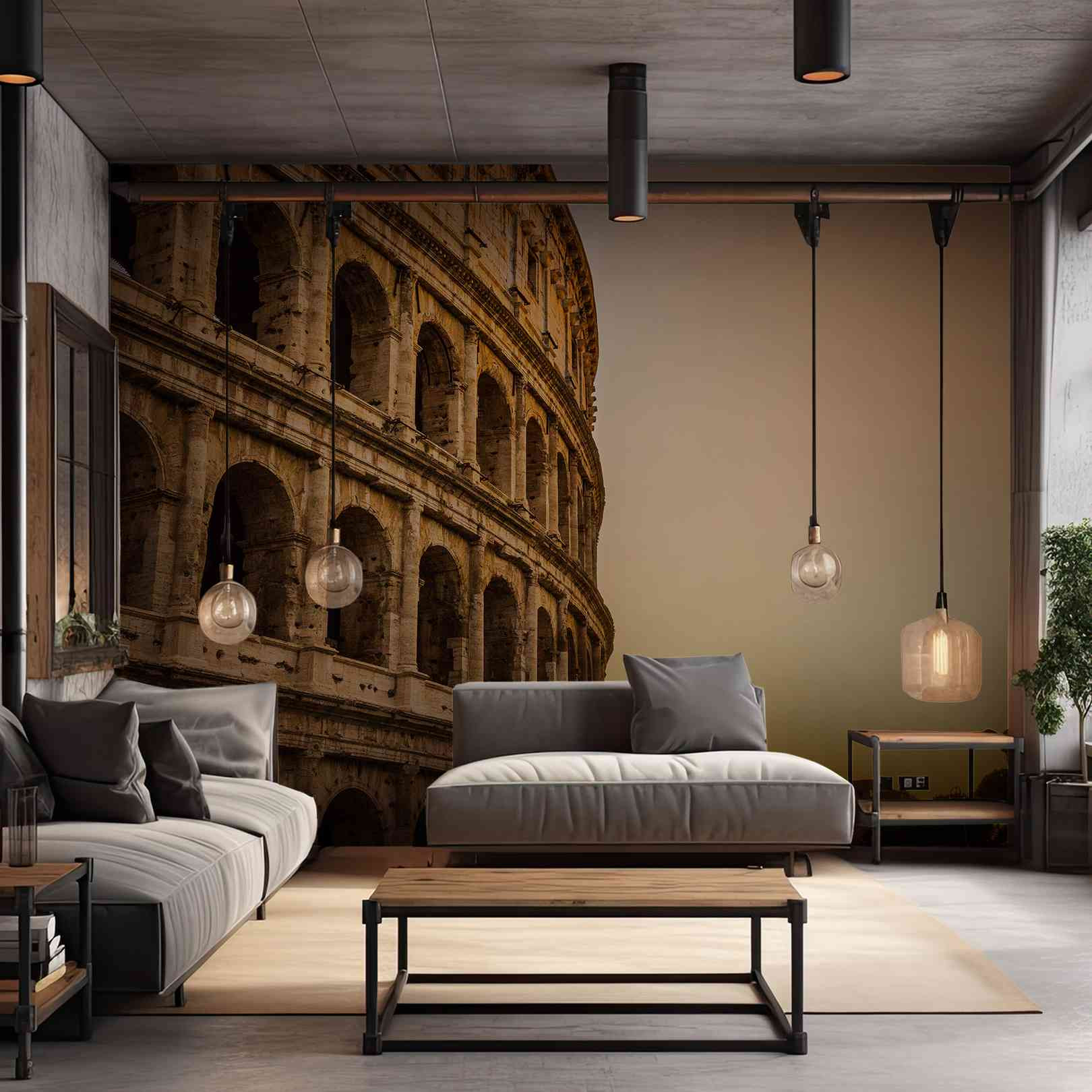The image depicts a meticulously designed living room with a modern industrial aesthetic. Dominating the left side of the room is a light gray sofa adorned with a perfectly arranged trio of pillows—light gray, dark gray, and brown. Central to the scene is a loveseat, also in light gray, accompanied by a single pillow. In front of the loveseat lies a horizontal coffee table with a light tan wood top and black metal piping, exhibiting the room's industrial motif. Both pieces of furniture are set on a matching gray area rug. The back wall strikingly features a large mural showcasing the side of the Roman Colosseum, adding a touch of historical grandeur. Hanging from the ceiling on long black cords are numerous decorative light bulbs, including three spherical ones and one shaped like a jar, contributing to the room's industrial appeal. The space is neat, organized, and clearly staged to present a clean and showy living area.